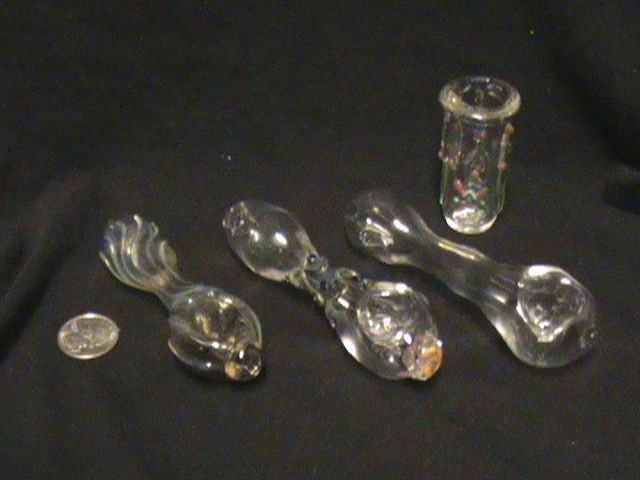In this seemingly color photograph, predominantly shaded in black and white tones, several glass objects are meticulously arranged on a slightly wrinkled black fabric cloth. The primary focus is on three glass pipes, likely drug paraphernalia, displayed diagonally from the top left to the top right of the image. Positioned from shortest to longest, the first pipe on the left features swirled designs and is accompanied by a quarter for scale, measuring approximately four quarters in length. The middle pipe appears smoother with a slightly textured front bulb, around five quarters long. The third and largest pipe, about four quarters in length, is smooth on both ends. Behind this largest pipe stands a tall, narrow glass cylinder, possibly a decorative or functional long tube. The light in the photograph casts from the left side, highlighting the intricate details and textures of the glass objects.